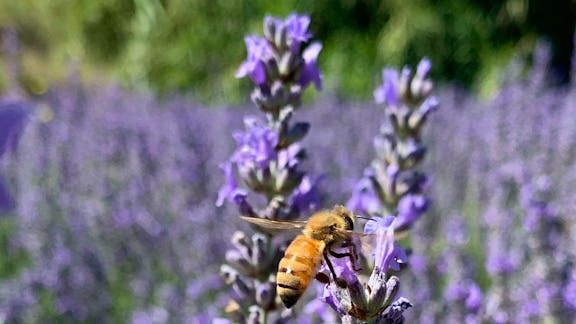In this vibrant nature photograph captured on a sunny day, a golden honeybee with distinct black stripes and outstretched wings hovers over a lavender plant, extracting nectar from its delicate purple petals. This highly detailed and hyper-focused wildlife shot features two additional lavender stalks in the foreground, framing the bee without detracting from it as the central subject. The background beautifully blurs into a tapestry of purple hues intermingled with patches of greenery, suggesting a lush field of lavender with perhaps a forest beyond. The image evokes a peaceful yet lively scene, highlighting the intricate details of the bee contrasted against a colorful, sunlit backdrop.